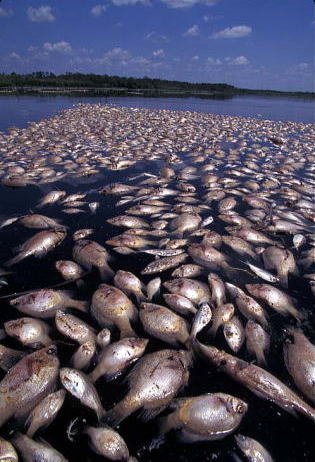In this photograph taken outdoors during daytime, we see a vast, serene body of water under a blue sky dotted with a few clouds. Hints of green from nearby trees and land appear in the background, enhancing the natural setting. However, the focal point of the image is a massive, unsettling sight: hundreds of dead fish floating at the surface. These fish, predominantly gray with some dark and pinkish hues, have their bloated bellies turned skyward, indicating they might have perished due to pollution, a red tide event, or a fish farming mishap. They are densely packed, stacked on top of one another, extending as far as the eye can see, creating a stark contrast against the otherwise peaceful aquatic scene. The photo captures this grim tableau in stark detail, making it a grisly snapshot of nature.